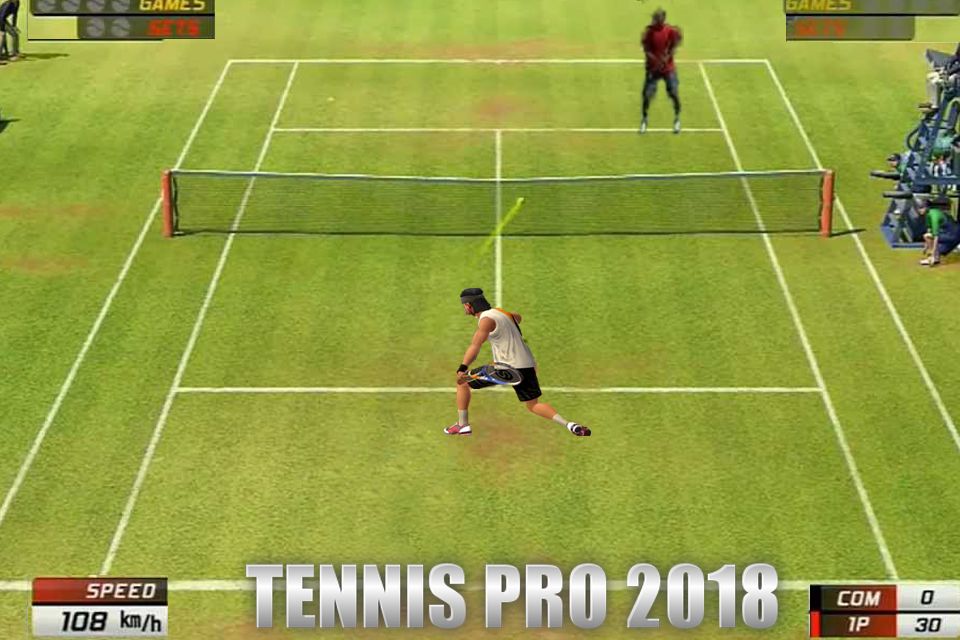The image is a screenshot from the tennis video game "Tennis Pro 2018," with a detailed view from behind one side of the court, showcasing singles play. At the top left and right corners, the screen tracks the games and sets for each player in yellow and red, respectively. The bottom of the screen prominently displays "Tennis Pro 2018" in grayish-white capital letters. Below that, in the bottom right corner, it shows the score: COM (computer) at zero and 1P (first player) at 30, indicating that the player is winning.

The foreground features a lighter-complexioned player wearing a white sleeveless shirt, black shorts, black shoes, and a headband with longer hair, just after hitting a lime-green tennis ball. This player's action resulted in a speed reading of 108 kilometers per hour, likely the service speed, displayed at the bottom. The tennis racket of this player is blue.

In the far court, a darker-skinned player with a blurry appearance wears a red shirt, gray shorts, and white shoes. Both players are engaged in the game, with distinctive clothing and positions described clearly. Additionally, the orange posts of the net and a chair umpire can be seen in the far-right side of the image. The visual elements and on-screen information indicate that this animated, somewhat dated-looking game is being played on a console or computer.